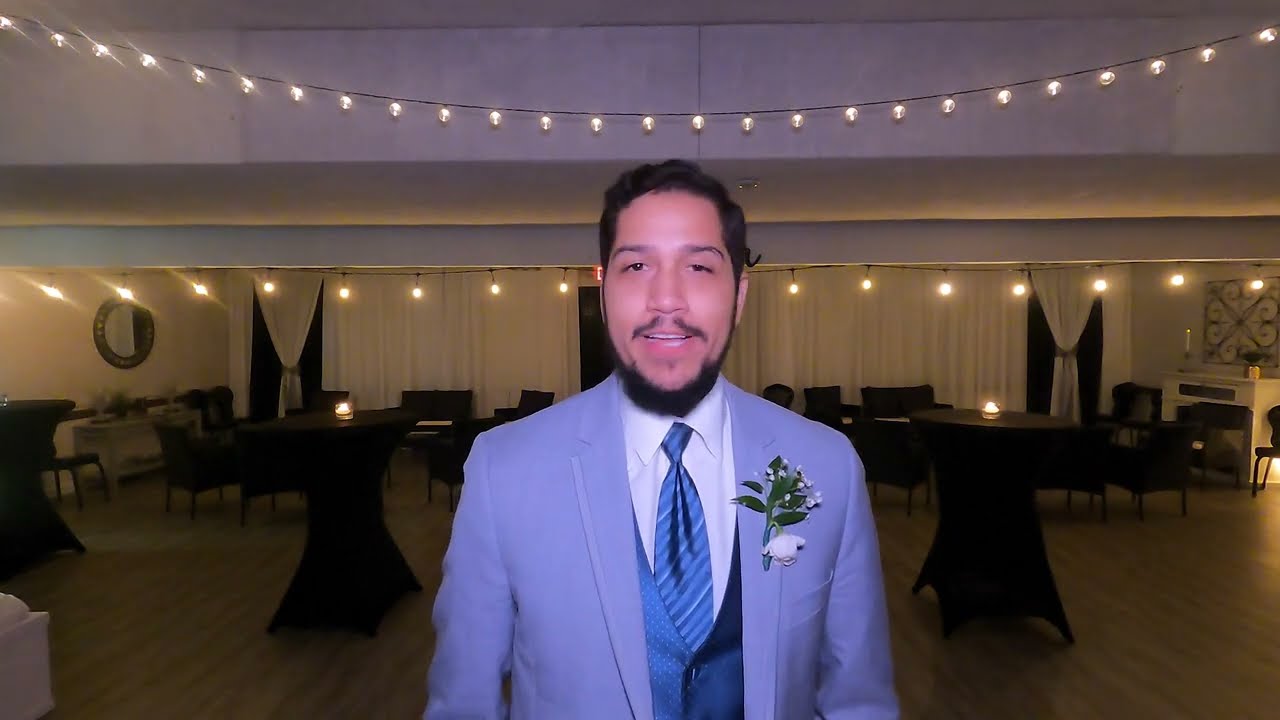In the center of the image stands a man who appears to be talking or smiling into the camera. He has short black hair and a black beard with a lighter mustache. The man is dressed in a light blue suit complemented by a matching blue vest, a darker blue striped tie, and a white button-up shirt. A green and white flower arrangement adorns his left breast pocket. He is situated in a dimly lit room that resembles a ballroom or conference center, with wooden floors and a variety of tables. The backdrop features several round, black standing tables, each with a candle, and more armchairs surrounding smaller tables further back. Behind him, white curtains cover the far wall, and a white fireplace with a tall pillar candle is visible on the right side of the image. The ceiling and wall lights add a warm, ambient glow to the otherwise empty formal dining area.